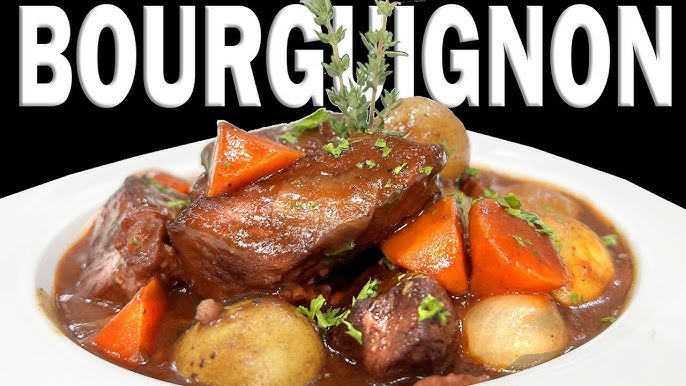In the foreground, a white dish contains a hearty serving of beef bourguignon, with the word "BORGUIGNON" prominently displayed in bold white letters against a dark black background. The dish features tender, brown-colored beef submerged in a rich, dark brown gravy. Nestled within are whole, round potatoes and sliced carrot chunks, all immersed in the savory broth. Green spices add a touch of color, with two sprigs standing upright and smaller green leaves scattered on top. The bowl itself is round with a notable ridge extending outward. The presentation captures the essence of a comforting and flavorful stew, promising a savory experience.